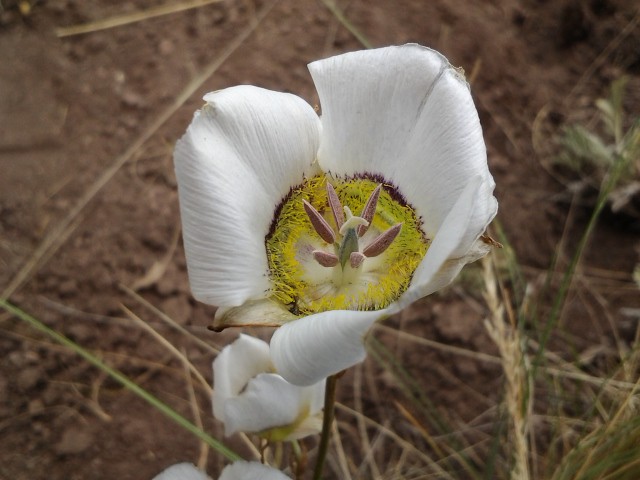The photograph showcases a striking white flower situated prominently against a backdrop of barren dirt, interspersed with dried grass and sparse green foliage. The flower's wide, curled petals frame an intricate central structure. This middle part is characterized by its pale greenish-yellow hue and is crowned with a peculiar, cactus-like formation. This formation is topped with a white segment that forks into three parts and is adorned with six small pink buds. Surrounding the main flower, there are hints of other blossoms peeking through the sparse vegetation, adding layers of depth to the desolate background. The overall composition captures the stark beauty and resilience of the flower in its harsh surroundings.